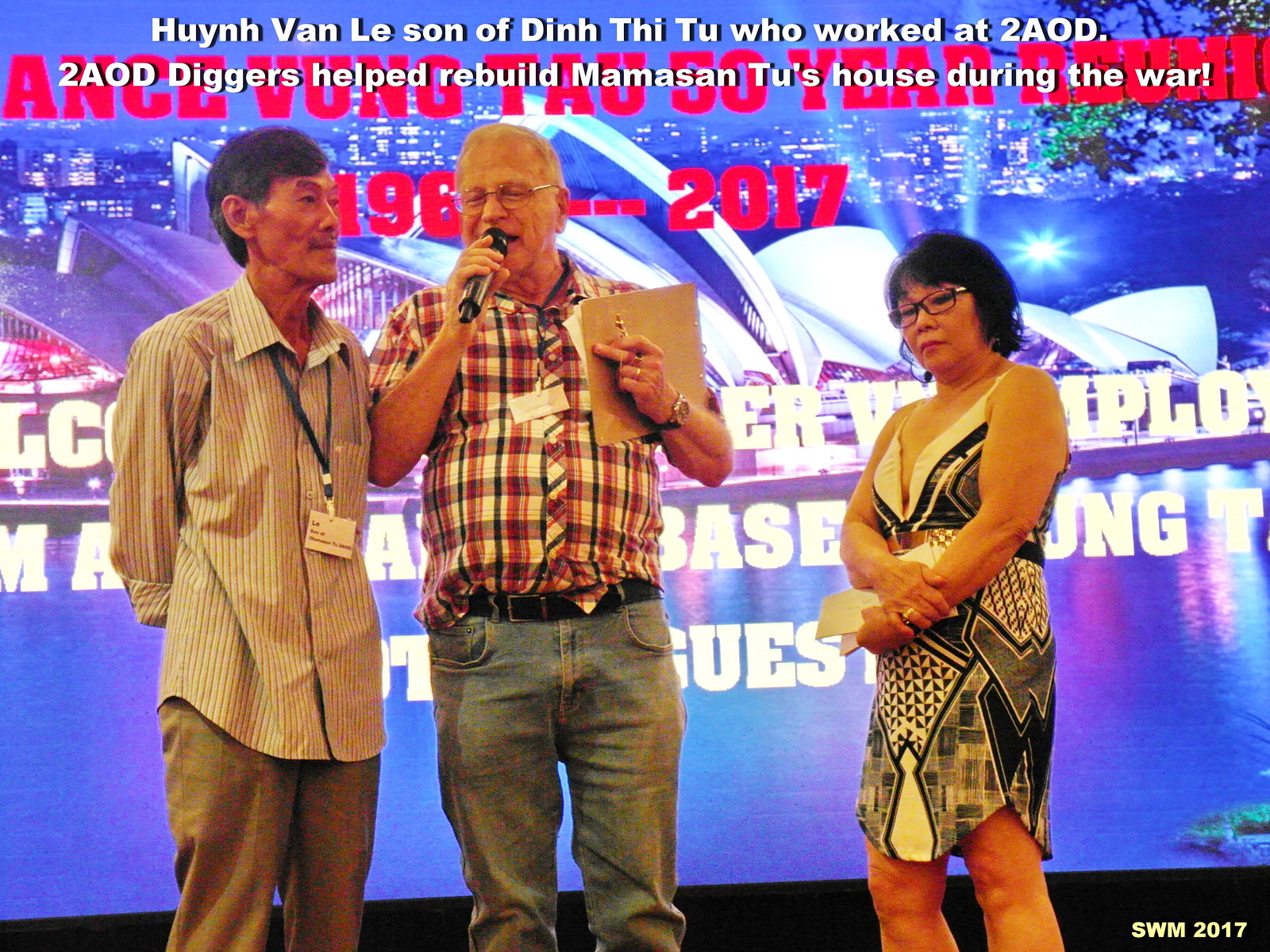In the photograph, taken inside a building with an amphitheater-like setting, a host is interviewing two people on stage. The host, positioned towards the left, is an older man wearing a white striped shirt and blue jeans, complemented by a blue lanyard and a tag. He is holding a microphone in one hand and a clipboard with a pencil in the other, while sporting a watch on his left wrist. To his right stands an older man with glasses, donned in a red and black checkered shirt. Further to the right is a woman with short black hair, glasses, and a black and gray dress. Behind them, the backdrop features an image of Sydney, Australia, and written in white font at the top, the text reads: "Hyun Van Lee, son of Din Thuty, who worked at 2AOD. Two AOD diggers helped rebuild Mama San Thu's house during the war." Additionally, "SWM 2017" is displayed in the bottom right corner. The scene is both vivid and detailed, capturing a poignant moment of commemoration and reflection.